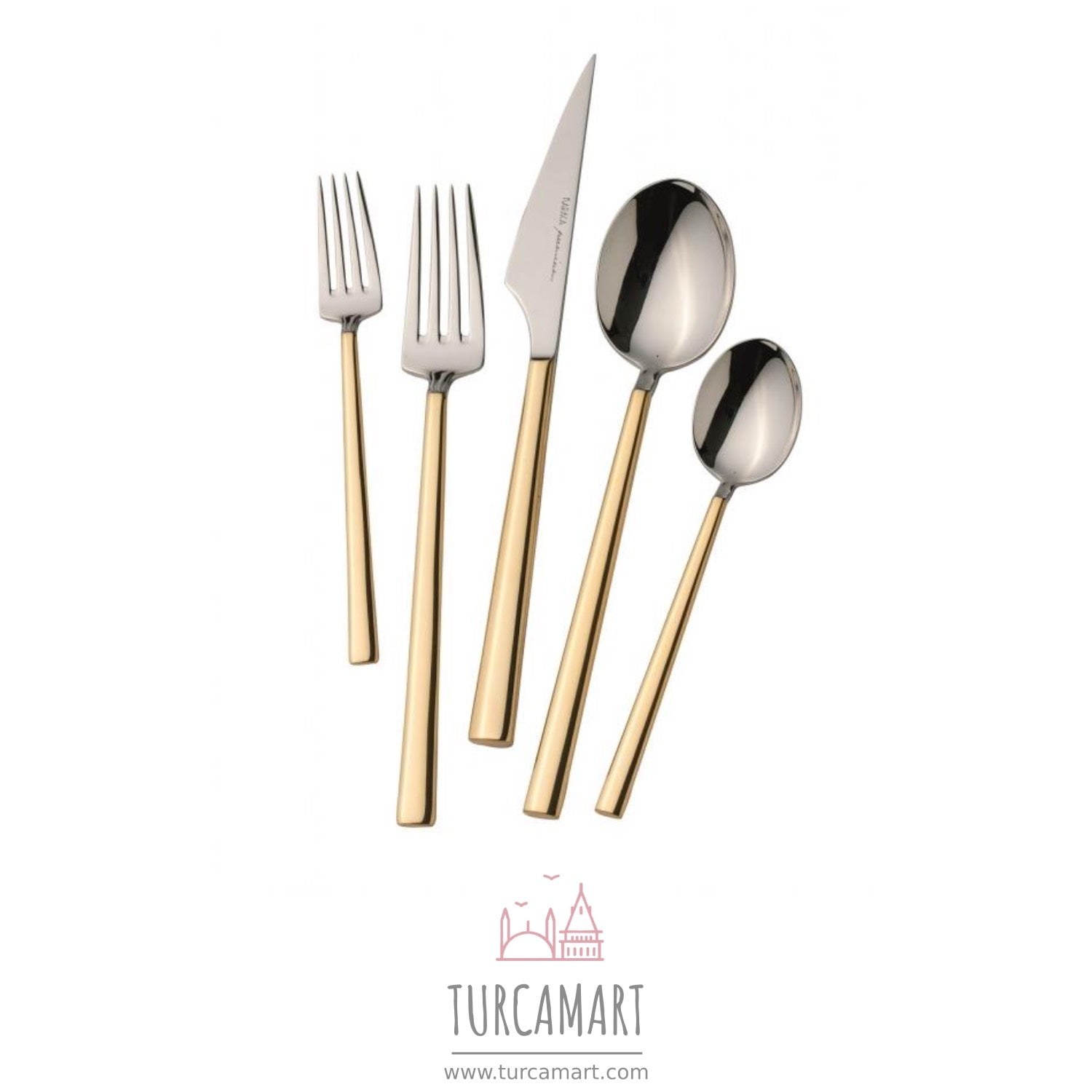The image displays a set of five pieces of cutlery neatly arranged on a clean, white background. Centered in the image are two forks, one shorter than the other, positioned to the left. To the right sits a silver knife with a gold handle. On the far right are two spoons, similarly differing in size, both featuring the same combination of gold handles and silver food-contact parts, giving them a sleek, modern look. At the bottom of the image, an illustration in red depicts two buildings with their pointed structures resembling a castle or mosque, accompanied by two birds flying overhead. Below this illustration is the text "Turcomart" with the URL "www.turcomart.com." This overall composition gives the impression of a digital, CGI-like advertisement for Turcomart cutlery.